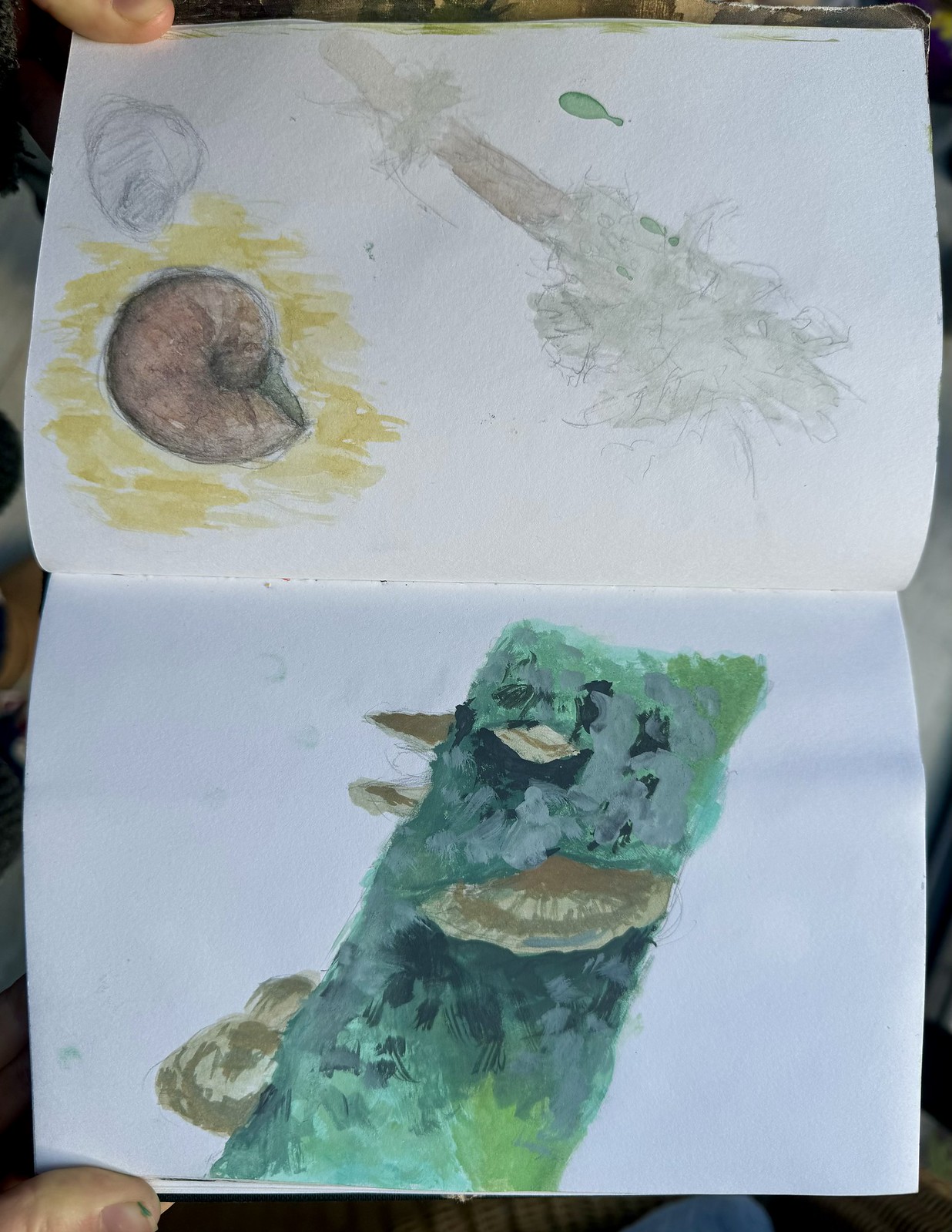The image portrays an open art journal showcasing intricate, mixed-media illustrations. The top page displays a brown snail shell set against a yellow background, accompanied by delicate, lightly drawn flora. This shell is spherical with a defined black outline. Adjacent to it is a branch with white sprouting leaves. The bottom page reveals a distinctly angular green bird, with accents of blue and light blue. Its rectangular body is complemented by a visible beak and eye. Additionally, a human thumb is seen holding the page in place, emphasizing the hand-crafted nature of the artwork. The journal appears to capture various elements of nature through a mix of media, including colored pencil, watercolors, and possibly charcoal. The overall composition is both whimsical and detailed, rendering a charming portrayal of natural scenes.